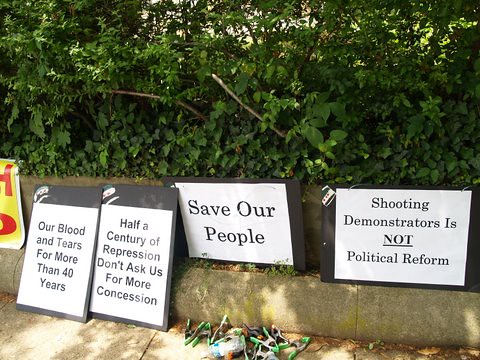This vivid photograph captures an outdoor scene in the middle of the day, showcasing a cement ground with a tan stone flooring and a curb just above it. There are no people in the image, but multiple black and white protest signs are laid out predominantly at the bottom of the photograph, with a green bush positioned above them. The signs convey powerful messages such as "Our blood and tears for more than 40 years," "Half a century of repression. Don't ask us for more concession," "Save our people," and "Shooting demonstrators is not political reform." The colorful backdrop includes hues of black, white, yellow, red, green, gray, and light green, enhancing the vividness of the scene. The absence of date or other contextual information focuses attention solely on the urgent pleas displayed in the signs.